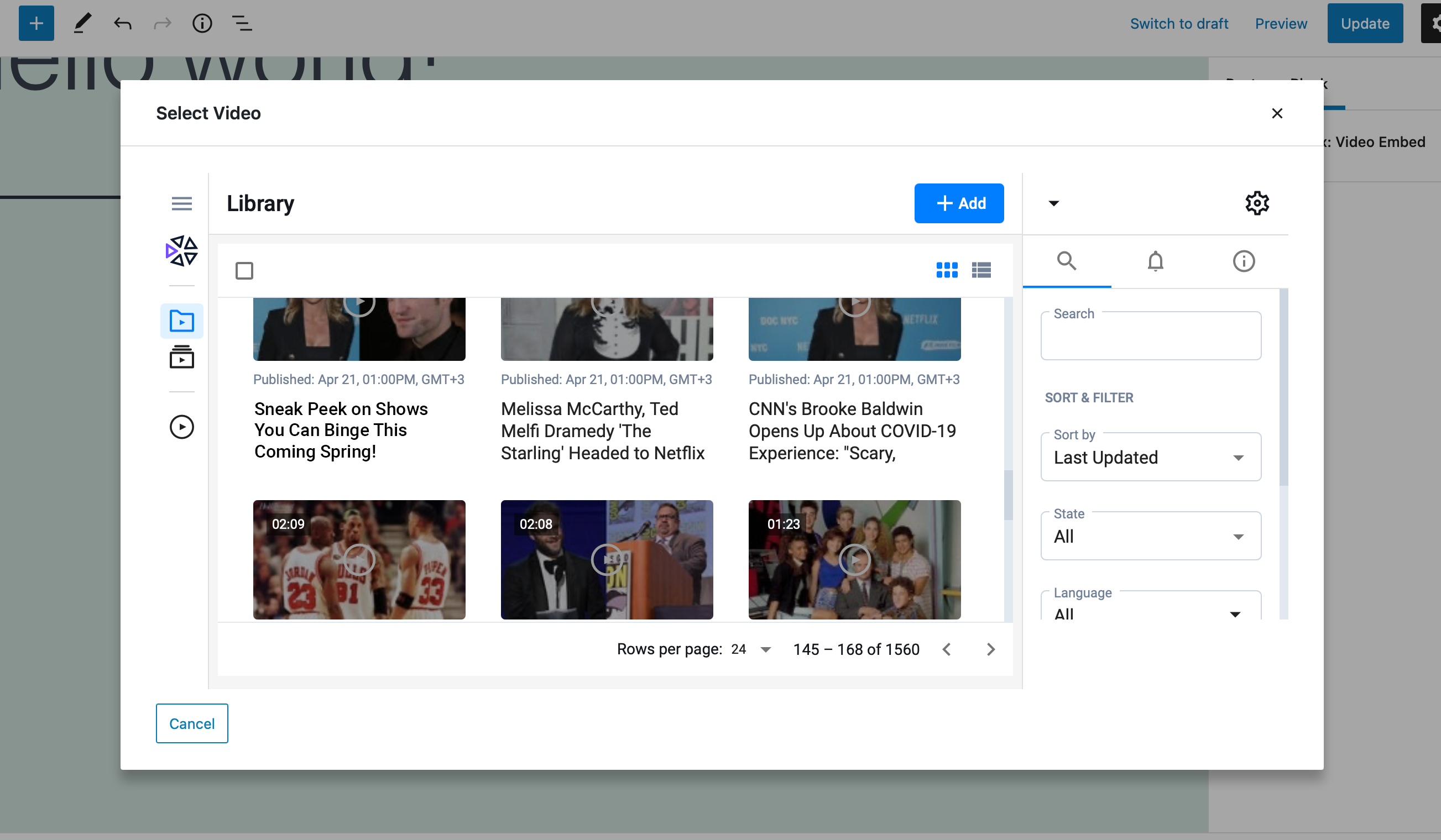This is a screenshot of a website with a prominent pop-up window in the center, which stands out against the grayed-out background of the site. The pop-up is a media selection interface titled "Select Video," and includes a library section. Within the library, there are six visible video thumbnails:

1. **Sneak Peek on Shows You Can Binge This Coming Spring**
2. **Melissa McCarthy, Ted Melfi, Dramedy, _The Starling_, Headed to Netflix**
3. **CNN's Brooke Baldwin Opens Up About COVID-19 Experience: Scary**

The titles of the remaining three thumbnails are partially cut off, though more videos can be browsed by scrolling. At the top of the pop-up, there's a blue icon with a plus symbol labeled "Add."

The lower section of the pop-up indicates pagination, showing "Rows per page: 24," and highlights the current range, "145 to 168 of 1560 videos."

On the right side of the pop-up, there are advanced search options including fields and filters for search queries, sorting by last updated, state, and language. Additionally, there are icons for notifications (bell), information (eye), and settings (cogwheel).

Due to the grayed-out background, the details of the main website are obscured, but it appears to be some sort of editor interface.